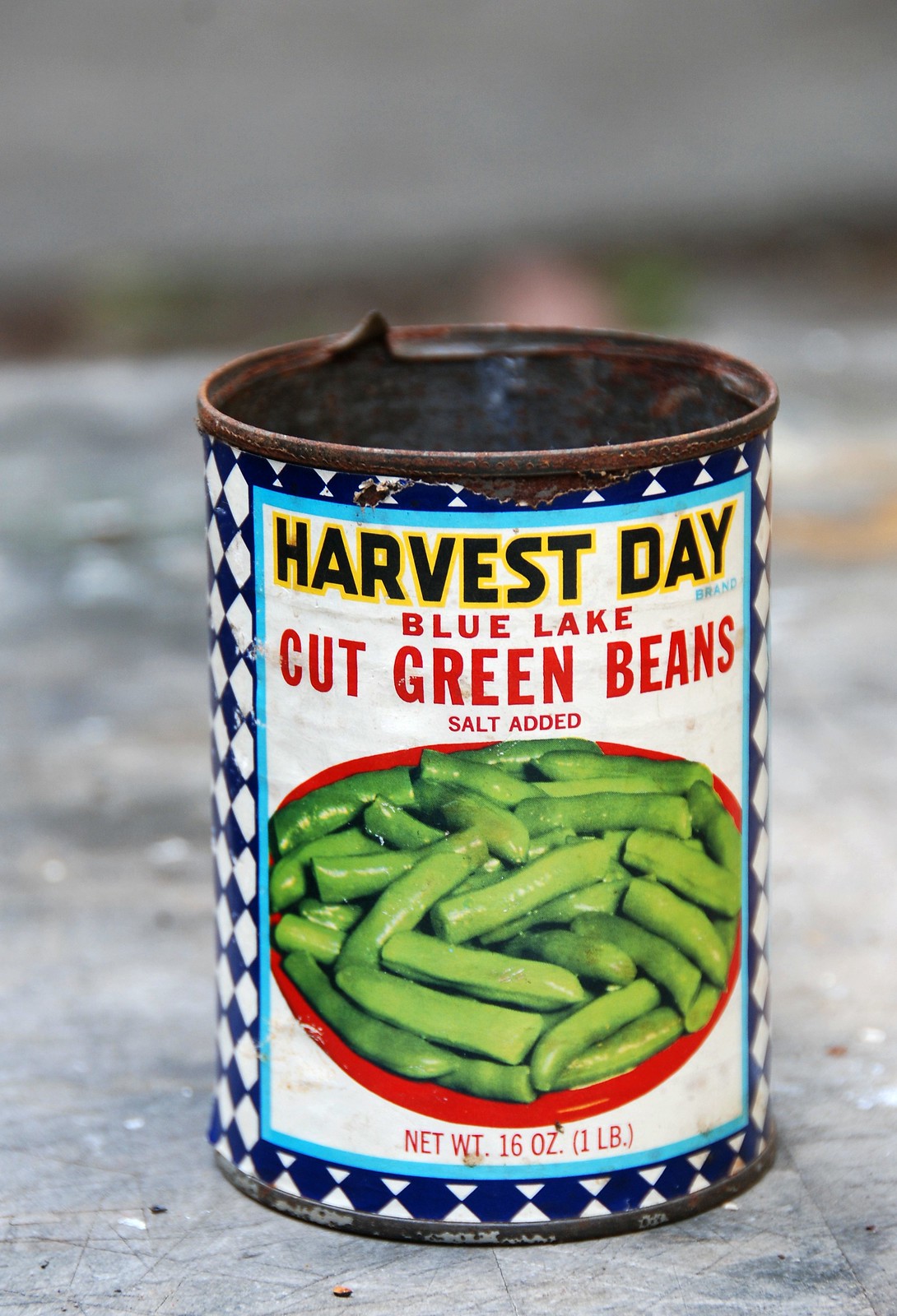The photograph showcases a tin of "Harvest Day" Blue Lake cut green beans with added salt. The label is primarily white, bordered by blue. The brand name "Harvest Day" is prominently displayed in bold black lettering, each letter outlined with a yellow border. Below this, the product description "Blue Lake Cut Green Beans" is written in red. A vivid image of the green beans arranged on a red plate is featured prominently on the label. The remainder of the label features a black and white diamond pattern, creating a striking visual contrast. The can rests on what appears to be outdoor concrete, and intriguingly, it seems to contain something black, rather than the expected green beans.